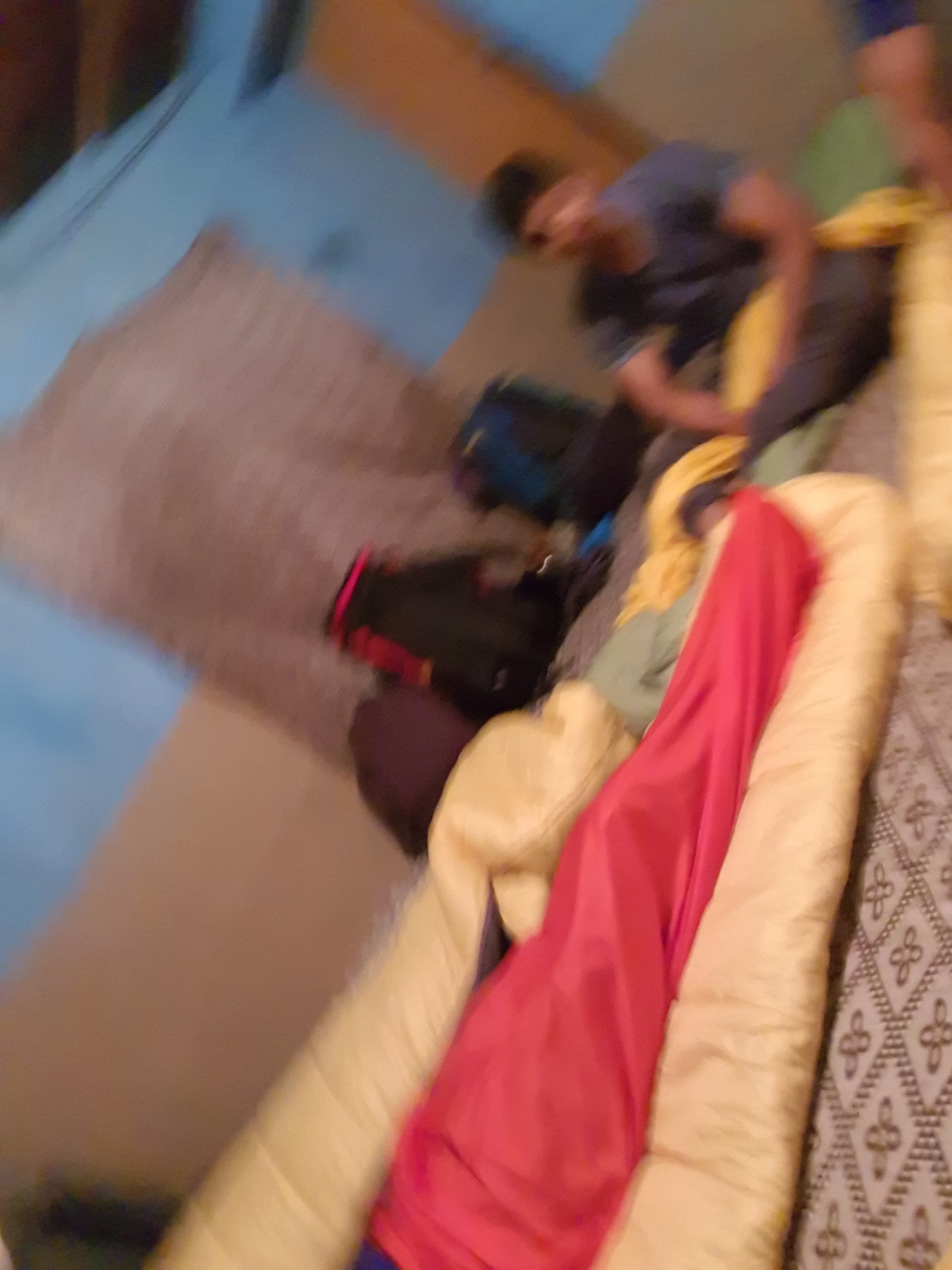The image depicts a cozy indoor setting featuring two gold sleeping bags laid out on a tan and brown patterned carpet. One of the sleeping bags appears to be occupied, with the visible figure wrapped in a luxurious, silky red satin blanket. Adjacent to this is another gold sleeping bag, whose occupancy is uncertain. At the foot of these sleeping bags, a man is seated on a bright lime green mat, partially covered by a gold blanket over his lap. The man, dressed in brown pants, obscures his hands under the blanket. In the background, several backpacks are propped against a wall, which is partially draped with a piece of brown material, seemingly serving to cover an opening. The overall ambiance suggests a warm and sheltered environment.